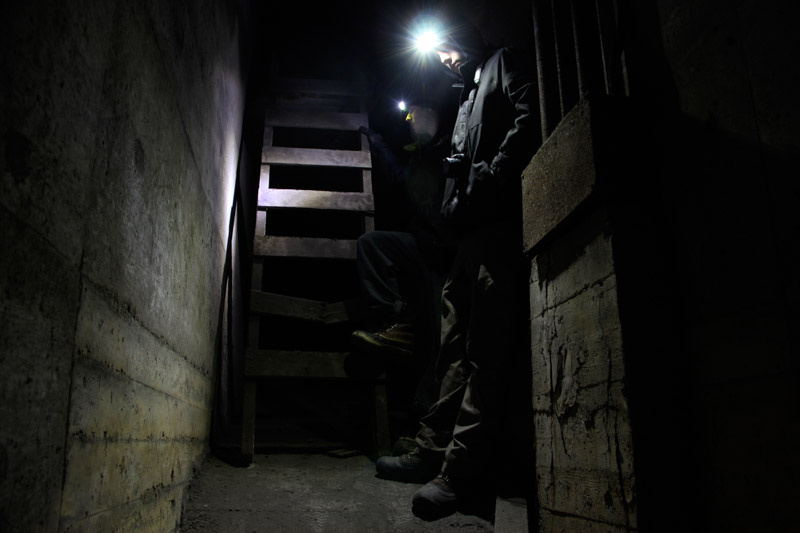In this dark and gloomy photograph, the setting appears to be an underground dungeon or basement with a damp, claustrophobic atmosphere. The walls and floor are constructed from gray concrete, enhancing the dungeon-like vibe. In the center of the image, two figures are visible, primarily illuminated by the headlamps strapped to their heads. The primary figure, dressed in black overalls, heavy work boots, and a black jacket, stands next to a rudimentary wooden staircase or ladder that descends into this confined space. He gazes curiously downwards, his face partially visible in the dim light. Another figure is partially visible behind him, distinguished only by the faint outline of a foot and another headlamp. The headlamps cast stark light beams against the concrete walls, emphasizing the eerie and constricted feeling of the space. The overall ambience of the photograph is dark, disturbing, and meticulously captured, evoking a sense of isolation and mystery.